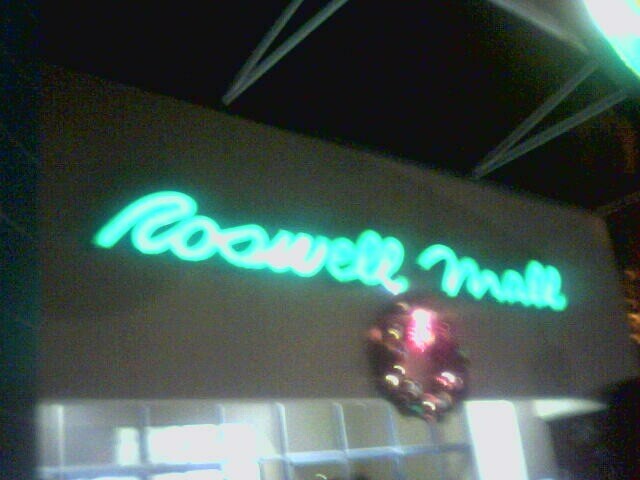The image shows the storefront of a shop named Roswell Made, which appears to specialize in clothing. The exterior of the store features a solid gray upper facade, prominently displaying the store's name, "Roswell Made," in elegant turquoise script. Adding to the festive ambiance, a beautifully decorated Christmas wreath, adorned with ornaments and illuminated accents, is displayed above the entrance. A vibrant red ribbon crowns the wreath, enhancing its holiday charm. The front of the store boasts large, floor-to-ceiling windows that offer a glimpse inside. The scene is set at night, with light from the store's upper signage casting a warm glow onto the adjacent parking lot.